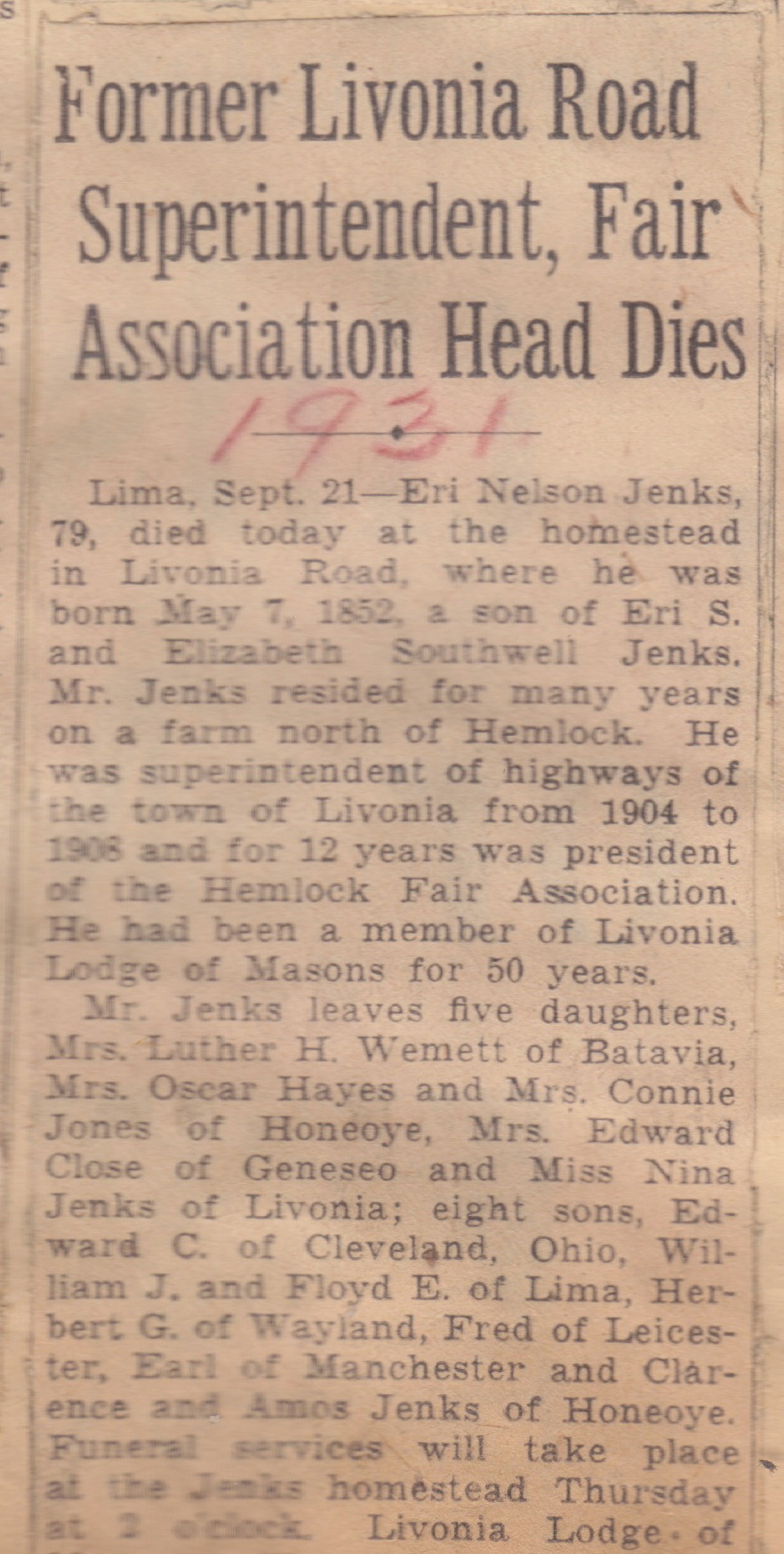The image features a scan or photograph of a cutout from an old newspaper obituary, its paper faded to a dark brown hue from its original white. The top part of the article bears the headline in black print: "Former Livonia Road Superintendent, Fair Association Head Dies." Above the article, "1931" is written in red pencil. The obituary begins with, "Lima, September 21. Larry Nelson Jenks, 79, died today at the homestead in Livonia Road, where he was born May 7, 1852, a son of Harry S. and Elizabeth Southwell Jenks." It details that Mr. Jenks lived on a farm north of Hemlock, served as the superintendent of highways for the town of Livonia from 1904 to 1906, and was president of the Hemlock Fair Association for 12 years. He was also a member of the Livonia Lodge of Masons for 50 years. The obituary lists his surviving family: five daughters—Mrs. Luther H. Wemmett of Batavia, Mrs. Oscar Hayes and Mrs. Connie Jones of Honeyoe, Mrs. Edward Close of Geneseo, and Ms. Nina Jenks of Livonia—and eight sons—Edward C. of Cleveland, Ohio, William J. and Floyd E. of Lima, Herbert G. of Wayland, Fred of Leicester, Earl of Manchester, and Clarence and Amos Jenks of Honeyoe. The funeral services were to be held at the Jenks homestead on Thursday at 2 o'clock. The lower part of the text is cut off.